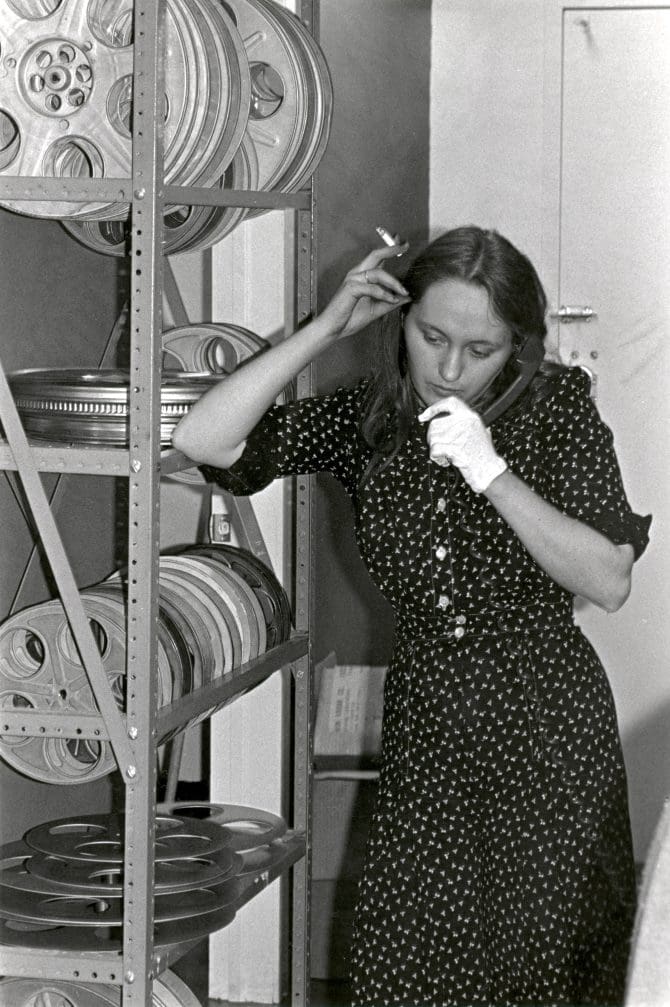In this black and white photo, a young white woman in her 20s or 30s with brown hair that falls past her shoulders is seen leaning against a steel shelf filled with old film reels and canisters. She’s clad in a black dress adorned with white polka dots or a small pattern and features buttons running down the front. Her dress’s sleeves reach almost to her elbows. She wears a white glove on the hand that holds a black telephone to her ear, while in the other hand, she holds a nearly finished cigarette. The shelves behind her, loaded with variously oriented film rolls—some upright, some lying flat—add a complex texture to the image. The background reveals a white wall with a door featuring silver locks, indicating an indoor setting. The grayscale tones enhance the vintage feel of the photograph, capturing a moment that’s both mundane and nostalgic.